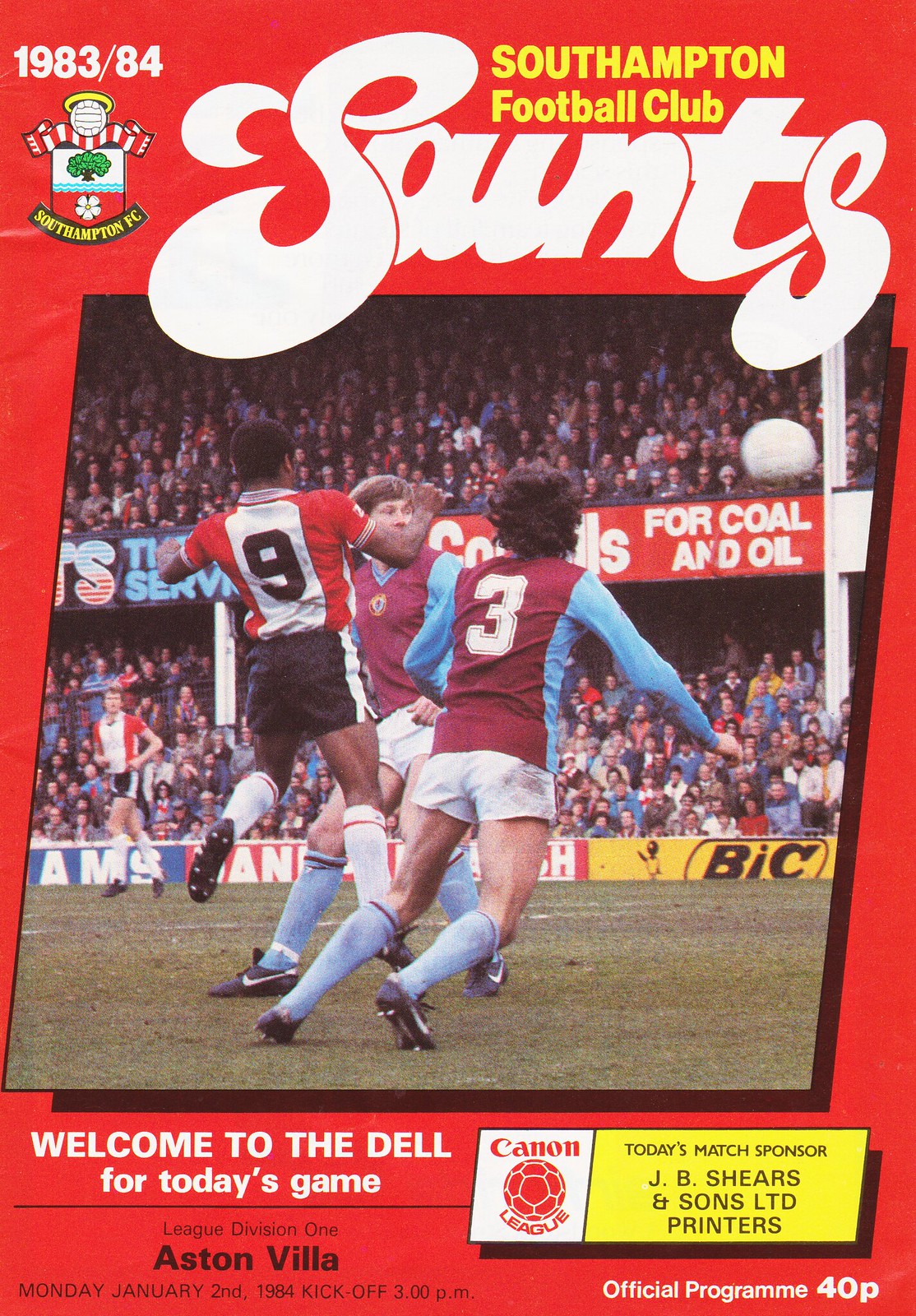This image is the weathered and grainy cover of a vintage soccer program poster for a game held during the 1983-84 season. Dominating the upper left is a red background emblazoned with white letters stating "1983-84" and "Southampton Football Club." Central to the design is a logo featuring a green tree, blue water waves, and a white flower, with a red and white muffler draped over a football at the top and "Southampton FC" curved above. Beneath this, the title "Saints" is prominently displayed in large, creative white fonts.

The central photograph captures three players in action on a grass soccer field, with two in maroon and blue jerseys, white shorts, and blue socks, and the third in a red and white jersey, black shorts, and white socks. The player in the blue and maroon jersey with the number three, and the one in red and white with jersey number nine, are seen battling for the ball in the upper right area of the image. Behind them, packed stands full of spectators can be seen, along with advertisements from sponsors like AMS, AN, and BIC.

Along the bottom border, the text "Welcome to the Dell for today's game" is displayed. Further details include "League Division 1, Aston Villa, Monday, January 2nd, 1984, kickoff 3 p.m." On the right-hand side, the program lists today's match sponsors: "Canon, JB Shears and Sons Limited Printers." To the bottom right, encased in a small box, it states "official program 40P."